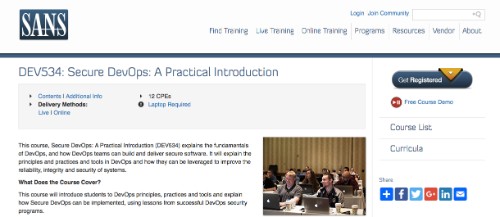Screenshot of a SANS Institute Website

The screenshot captures the homepage of the SANS Institute website. In the top left corner, the SANS logo is prominently displayed in white lettering within a blue rectangle. Spanning the right side of the header are several navigational tabs: Find Training, Live Training, Online Training, Programs, Resources, Vendor, and About. Above these tabs is a search bar accompanied by Login and Join Community options on its exterior.

Directly below the navigation bar is a horizontal blue divider which separates the header from the main content. The main content begins with a prominent title in blue lettering. Beneath this title, a gray box houses a series of hyperlinks in blue and black text.

Further down, the content area is structured into two paragraphs, each delineated by a title line. Adjacent to these paragraphs, on the right side, is an illustrative image depicting people working on computers.

On the far right side of the image, there is a dedicated section for sharing the webpage via various social media platforms, featuring numerous icons and links for seamless social connectivity.